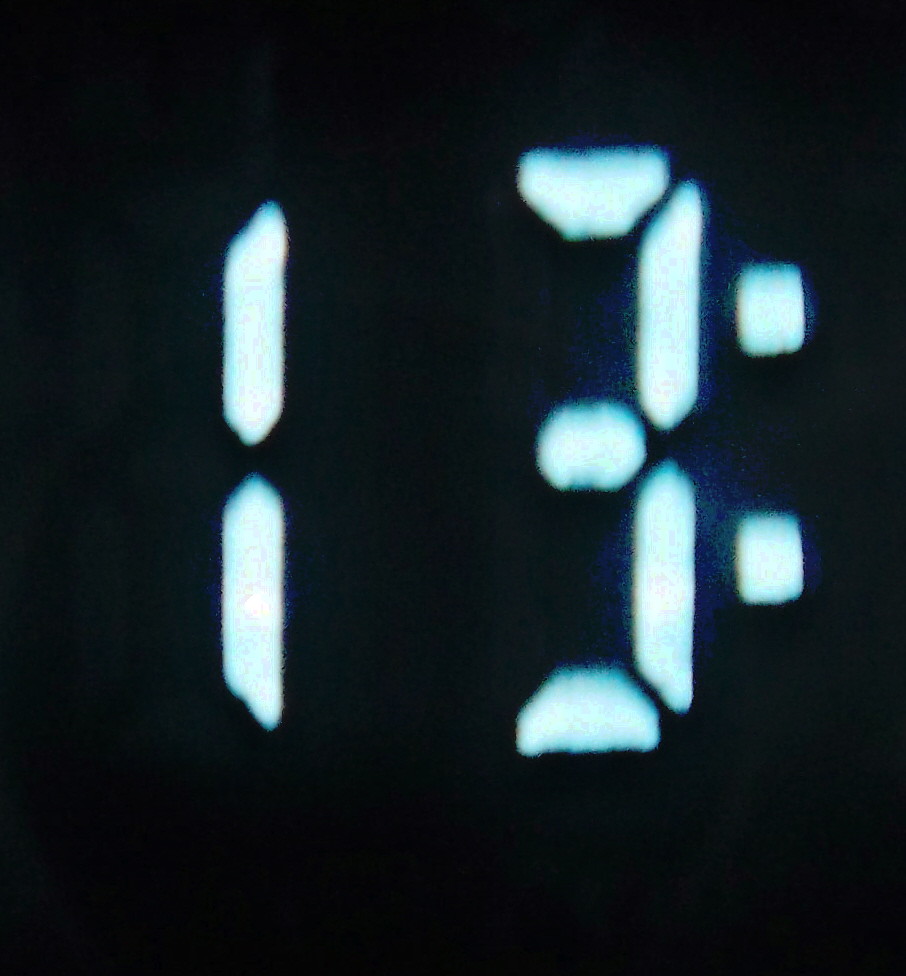This close-up photograph captures a digital alarm clock displaying the digits "13" against a solid black background. The numbers, illuminated in a stark white with a subtle light blue tint, stand out prominently due to the high contrast between the bright digits and the dark backdrop. The image is tightly focused on the clock's display, offering an almost abstract and minimalist aesthetic centered on these glowing figures.